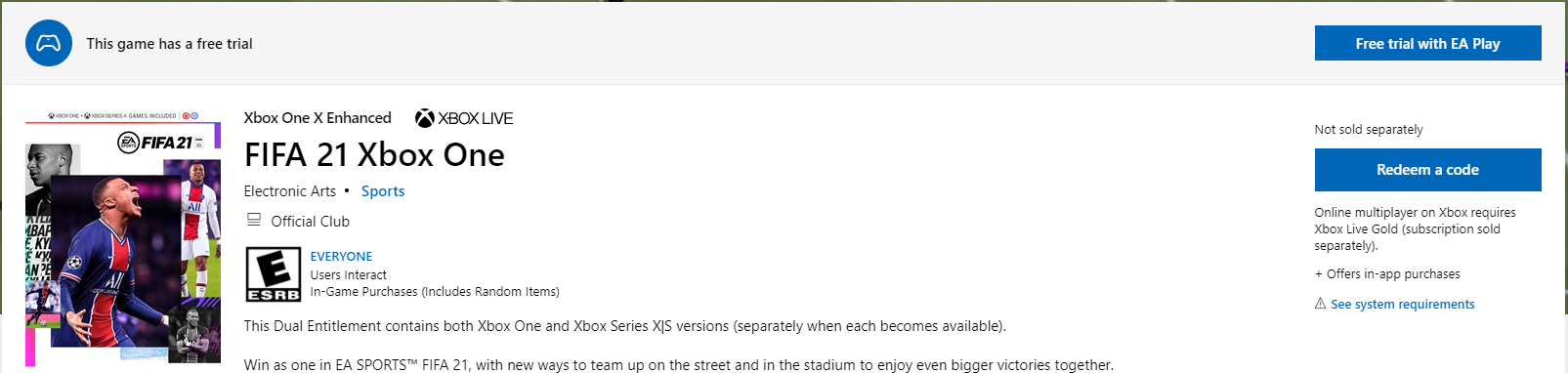This cropped screenshot features the EA Play website interface. Dominating the top right corner is a prominent blue button labeled "Free Trial with EA Play." In the top left corner, there's a blue circle containing a white game controller icon. Directly adjacent to the icon, text reads "This game has a free trial."

The background of the page is predominantly white. In the top left section, a thumbnail of the FIFA 21 box art is displayed. To its right, small black text indicates "Xbox One Enhanced," with the Xbox Live logo situated slightly further to the right, also in small black typography.

Prominently below these elements, the title "FIFA 21 Xbox One" is written in bold black letters. Underneath this title, in smaller black text, the publisher's name, "Electronic Arts," is listed. Towards the right of this, the genre "Sports" is identified in small blue font, while "Official Club" is presented in small gray letters underneath.

Towards the bottom left of the image, the game’s rating is indicated with an "E for Everyone" label. To the right of this label, "Everyone" is written in small blue font. Beneath this, a disclaimer in tiny print informs users that the game features "Users Interact with in-game purchases." Below this disclaimer lies a brief description of the game.